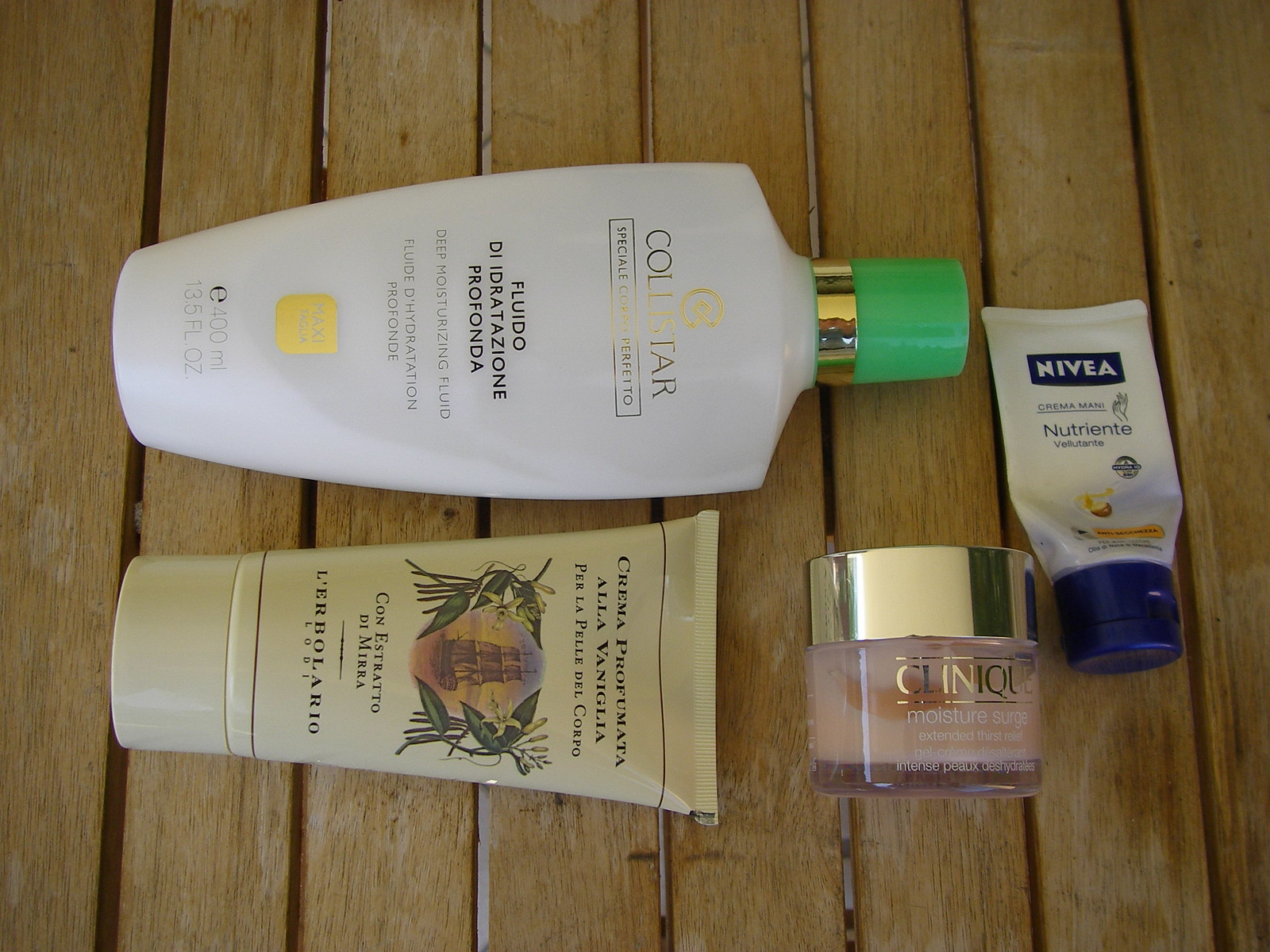This close-up aerial photograph captures four essential elements of a makeup routine displayed on a wooden table. The table, constructed of slats about two inches wide, features a light and dark brown wood texture. The topmost item in the image is a cream-colored bottle with a green lid and a white band around its neck. The text on the bottle suggests it contains a hydrating or deeply moisturizing fluid, possibly from a brand related to colt hair or a similar name.

Below this, a beige-colored tube adorned with a vintage illustration of an old ship flanked by leaves and flowers is visible. This tube contains an extract of some kind. 

Further down, on the left side, sits a small Clinique bottle, designed as a moisturizer in a skin-tone shade and capped with a gold lid.

Lastly, the composition includes a small tube of Nivea cream nutrient, characterized by its white body and blue lid. All these items rest elegantly on the wooden slats, inviting a closer look at the details of each product within the makeup ensemble.